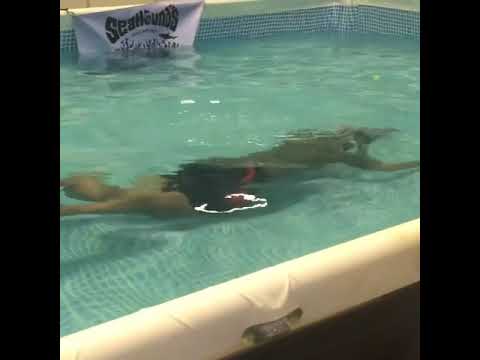The image depicts a narrow swimming pool viewed from the side, framed by white borders along both the left and right edges. The water appears to be an aqua blue, slightly tinged with green. The pool is likely not an in-ground type, hinted at by the foam-like structure of the border. Above the waterline, there's a visible light blue tile backsplash with tiny tiles. In the pool, which has an aqua blue color, swims a person wearing black swimming trunks with possibly red accents; their identity is not entirely clear, but they seem to be a man of Caucasian descent. This individual is submerged and swimming towards the far end of the pool, in a northeast direction. Toward the far background, partially submerged and hanging into the water, there is a white banner with black text, seemingly related to "Seattle Unns," although the full text is obscured. The photo captures a detailed view of the edges, water, swimmer, and the banner within the indoor pool setting.